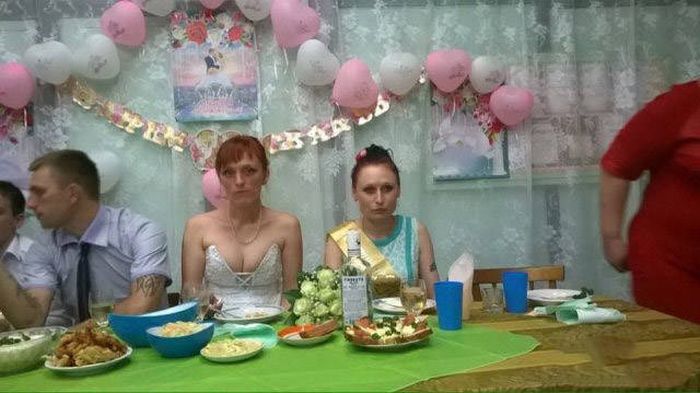The image depicts a lively celebration, likely a wedding, characterized by a joyful yet slightly somber atmosphere. Central to the scene is a dining table partially covered by a green tablecloth, adorned with an array of dishes including a plate of bread, chicken, and a dip, along with blue cups and a bottle of what appears to be alcohol. A bouquet of roses sits prominently in front of a woman. Heart-shaped balloons form an arch over the table, leading the eye to a sheer floral white curtain that spans the background. Above this curtain, there are small photos of a couple, presumably the bride and groom. A banner with indiscernible text stretches across the curtain.

Seated at the table are two men on the left, both gazing off-screen, and two women on the right, one wearing a possible wedding gown with visible cleavage and a pearl necklace, and the other in a purple and white dress with a gold sash and a tattoo on her left arm. Both women's expressions appear somewhat discontented. To the far right, a figure in a red full-length dress or shirt is partially out of frame, possibly having stood up from their seat.

The scene is rich with colors such as white, pink, green, blue, yellow, purple, red, and brown, enhancing the festive yet intimate ambiance.